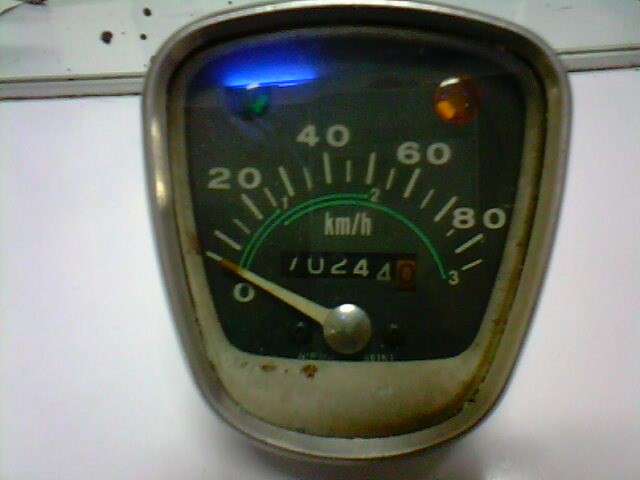The image depicts a detailed automotive dashboard gauge. The upper portion of the gauge, labeled "KM/H"—indicating kilometers per hour—features numerical markings at 20, 40, 60, and 80, interspersed with white lines, suggesting speed increments. A silver metal needle with a red tip currently points towards the indicated scale.

Directly below this main speedometer is a secondary, smaller gauge with green markings labeled 1, 2, and 3. This likely indicates a different measurement, such as fuel levels or RPM. The lower section also contains an odometer, showing the vehicle's total distance traveled. The odometer displays the numbers, possibly reading 70244, with the last three digits being more clearly visible as "024". These figures appear on a rolling mechanism that updates as the vehicle moves.

The entirety of the gauge setup is encased in a silver metal frame with a protective glass cover, which not only adds to the aesthetic appeal but also serves to keep out dust and debris.